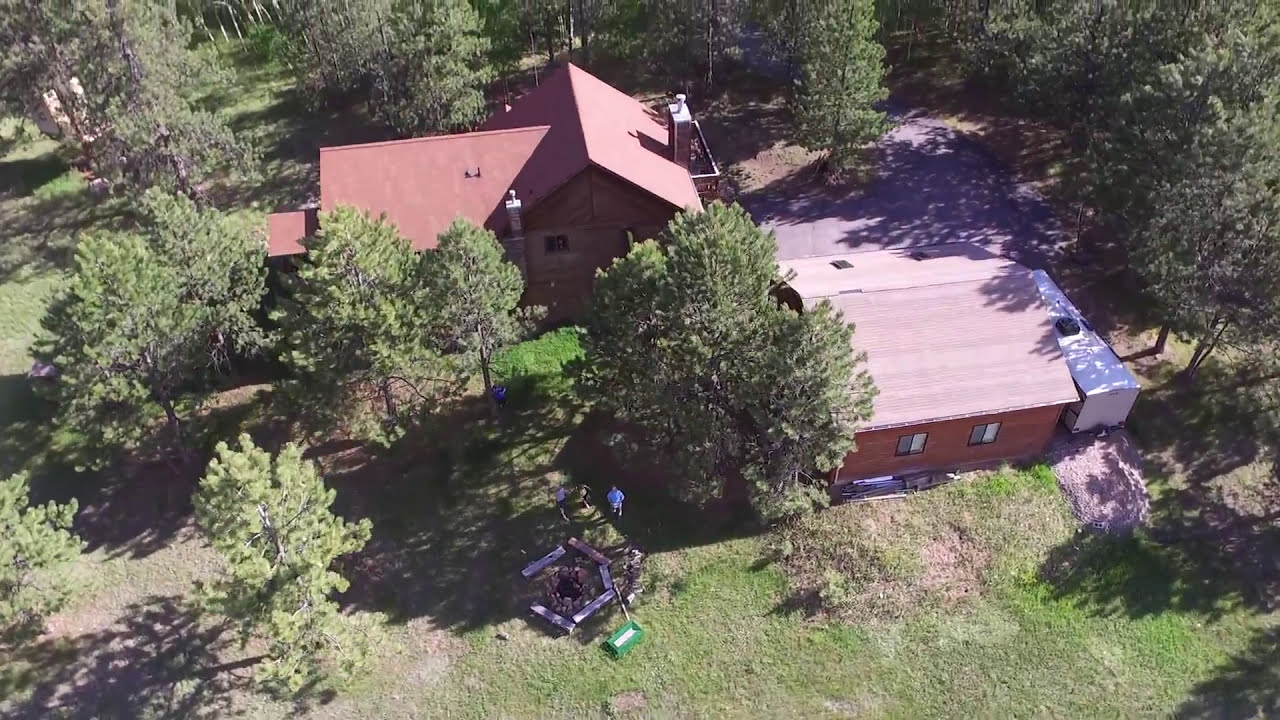This is an aerial view capturing two distinct houses set amidst a dense forest. The focal point is a multi-story house with a dark orange, steeply arched metal roof, and a brick exterior. The house features a prominent chimney with a silver-colored pipe extending from it. Trees and patches of grass surround the entire scene. 

To the right of this main house, there is a smaller, arched building with a light orange-red hue and two visible windows. Beside this smaller building is a white trailer, which has a brown circular item placed on its top. The trailer's hitch faces the camera.

In the bottom center of the image, two people are seen standing on the grass, under the shadow of nearby trees. They are positioned near a circular arrangement of five elongated structures, which appear to be forming a flowerbed. Adjacent to them is a dark green metal object featuring a light white strip in its center.

The overall landscape includes a mix of varying tree heights and conditions, creating a picturesque, well-manicured setting complemented by a secluded, tranquil atmosphere.